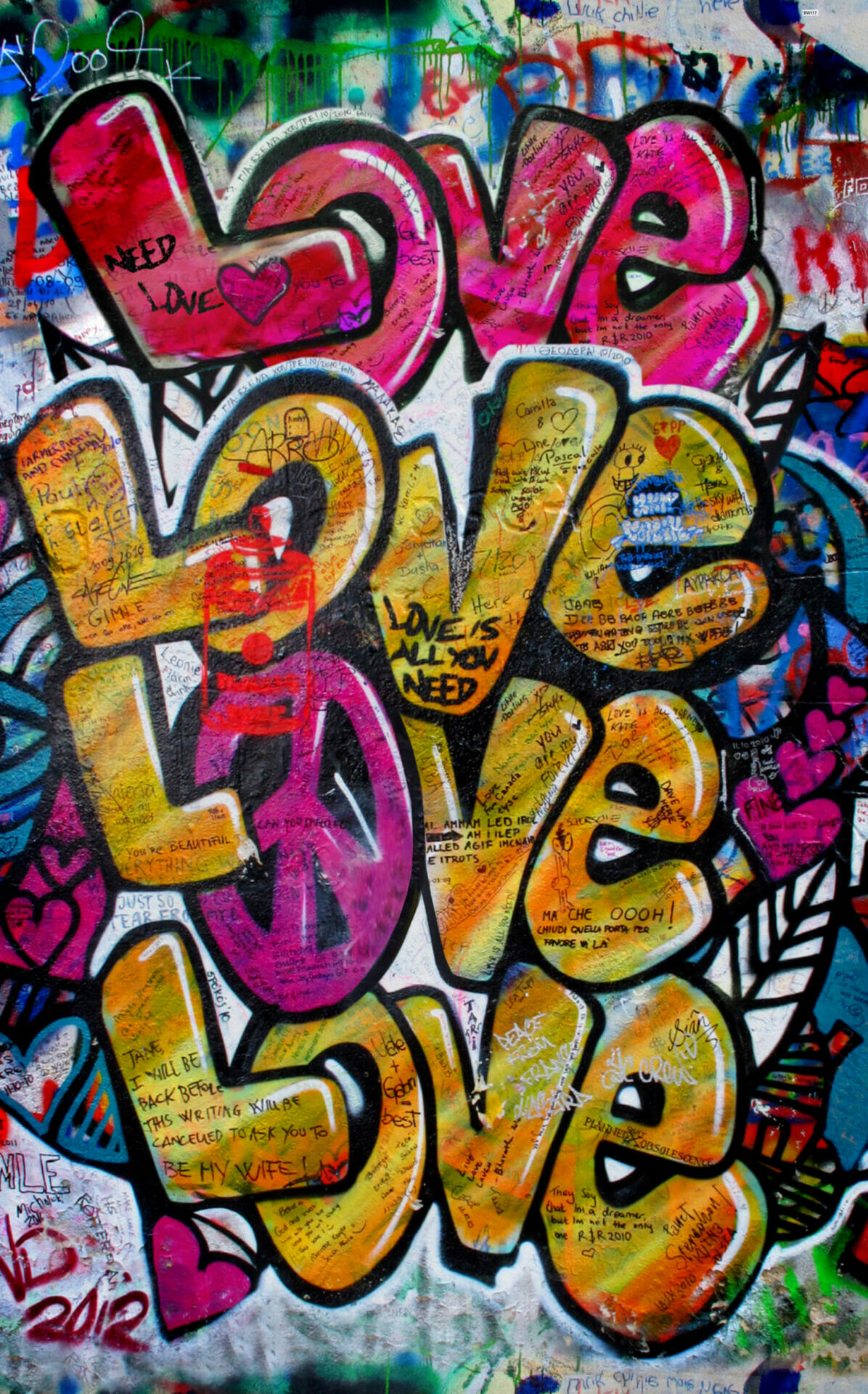In this photograph, an eye-catching piece of graffiti art prominently features the word "LOVE" repeated four times in bold bubble letters, stacked vertically. The topmost "LOVE" is rendered in vibrant pink and magenta, with red accents and white highlights adding depth and a bubbly texture. This word is outlined in thick black, with the L overlapping the O significantly, and the V and E squished together. Below this, the second "LOVE" is done in bright yellow and is filled with various doodlings and writings created with pens and markers from different sources. 

The third instance of "LOVE" showcases a unique twist where the O is replaced by a pink-magenta peace symbol. This version incorporates a blend of yellow, green, and orange hues, and like its predecessor, it is adorned with scribbles within the letters. The bottom "LOVE" repeats the multicolored theme, mixing yellow, orange, red, and green applied in a random splotchy pattern. This lower section also continues the motif of internal scribbles and doodles.

Surrounding these words, the background features thick black outlines depicting shapes such as hearts and feathers, as well as some indiscernible drippy graffiti. Additional colorful elements include purple and pink hearts scattered above and below the stack of words. At the very base of the image, light blue and white backgrounds frame the area, with “2012” written in purple text on the left-hand side. Scattered throughout the piece, one can also find text like "LOVE IS ALL YOU NEED" within the center of the V in the multicolored words, and "NEED LOVE" accompanied by a heart on the L of the top pink “LOVE.” This lively and vibrant graffiti mural encapsulates a message of love through a mix of vivid colors and diverse artistic expressions.